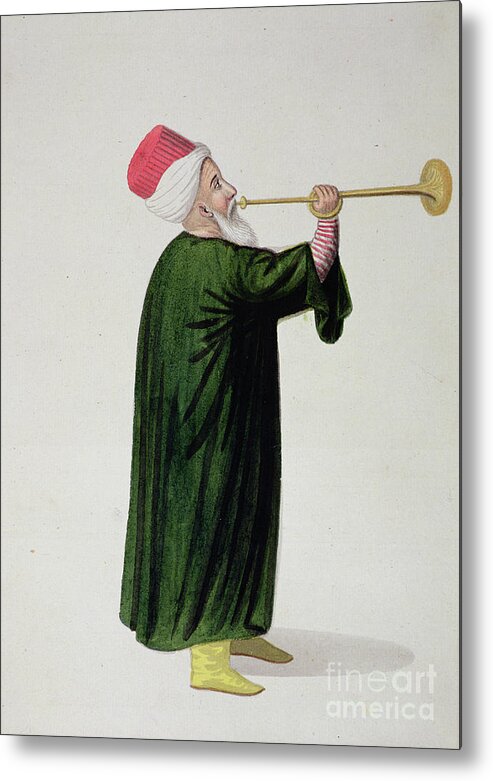In this detailed painting on a clean white background, an elderly Caucasian man is depicted in the midst of playing a long, thin brass or golden horn that he holds up to his lips with his right hand. His attire consists of a flowing, textured green robe, possibly made of corduroy or velvet, over a shirt with red and white stripes. His footwear is a pair of yellowish-brown, possibly gold, shoes that peek out from beneath his robe. The man, characterized by his white complexion and long white beard, wears a distinctive hat that features a red top and white bottom, reminiscent of a head wrap or turban. There are no textual elements within the painting itself, although it's noted that "Fine Art America" is inscribed at the bottom right corner. This image, rich in color and texture, is a drawn piece of art rather than a realistic photograph.